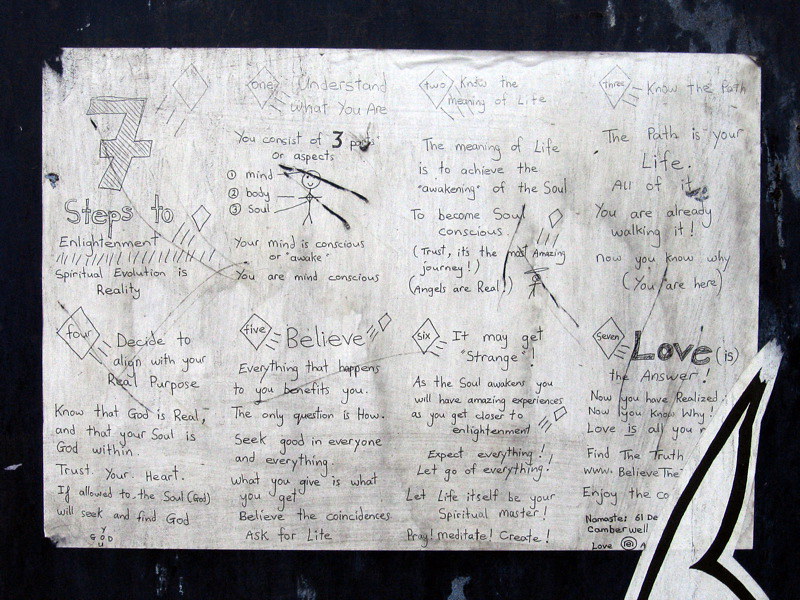The image depicts an open white notebook, filled with detailed handwritten notes and sketches using pencil. In the upper left corner of the left page, a prominent number "7" introduces the text "Seven Steps to Enlightenment" in elaborate, doodle-like letters. These steps are methodically listed from one to seven, with each number written out in words and accompanied by diamond-shaped bullet points. The steps cover themes such as "spiritual evolution is reality," "understand," "know the path," "believe," and culminate in "love." The lower right corner of the opposite page reiterates the notion with the phrase "Love is the answer." Although the text is a bit smudged in places, it captures a coherent spiritual theme. The notebook rests on a dark, partly ink-spotted surface, adding a raw, contemplative mood to the overall presentation.